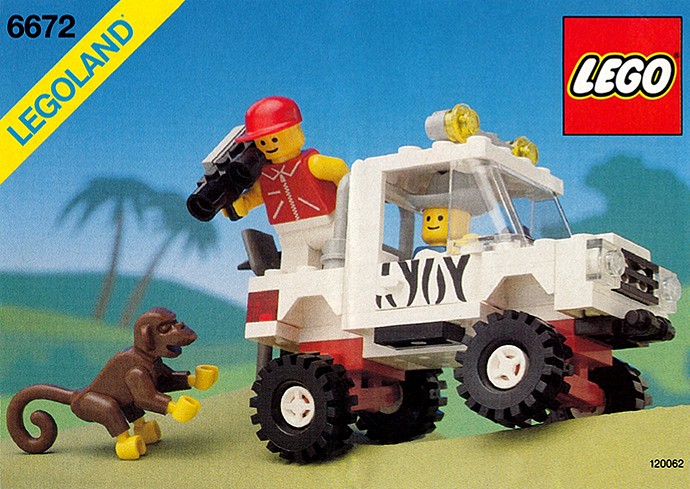This image appears to be a computer-generated, possibly promotional, depiction of a vintage LEGO toy set box. The image has a grainy quality and exhibits an old-school aesthetic. 

At the top left-hand corner, the number 6672 is displayed prominently in black letters. Directly beneath this number, a yellow-bordered blue banner reads "LEGOLAND." On the top right-hand corner, within a red rectangular area, the word "LEGO" is written in white letters.

The central focus of the image is a LEGO jeep, colored white with black and red accents, situated on the right side. The jeep features two LEGO characters: one with a red baseball cap standing in the back, wearing a white outfit with a red sleeveless shirt, holding a video camera and staring down at a LEGO monkey. The monkey, positioned in the bottom left-hand corner, is dark brown with yellow hands and feet. The other character, who has a grey cowboy hat, is behind the wheel of the jeep. Both characters are yellow, with black dots for eyes and a simple black-lined mouth.

The scene is set in a jungle-like environment, with greenish-brown sand beneath the jeep and blurred background elements including trees, green grass, and a blue sky. The overall composition gives a sense of playful adventure in a LEGO-themed world.